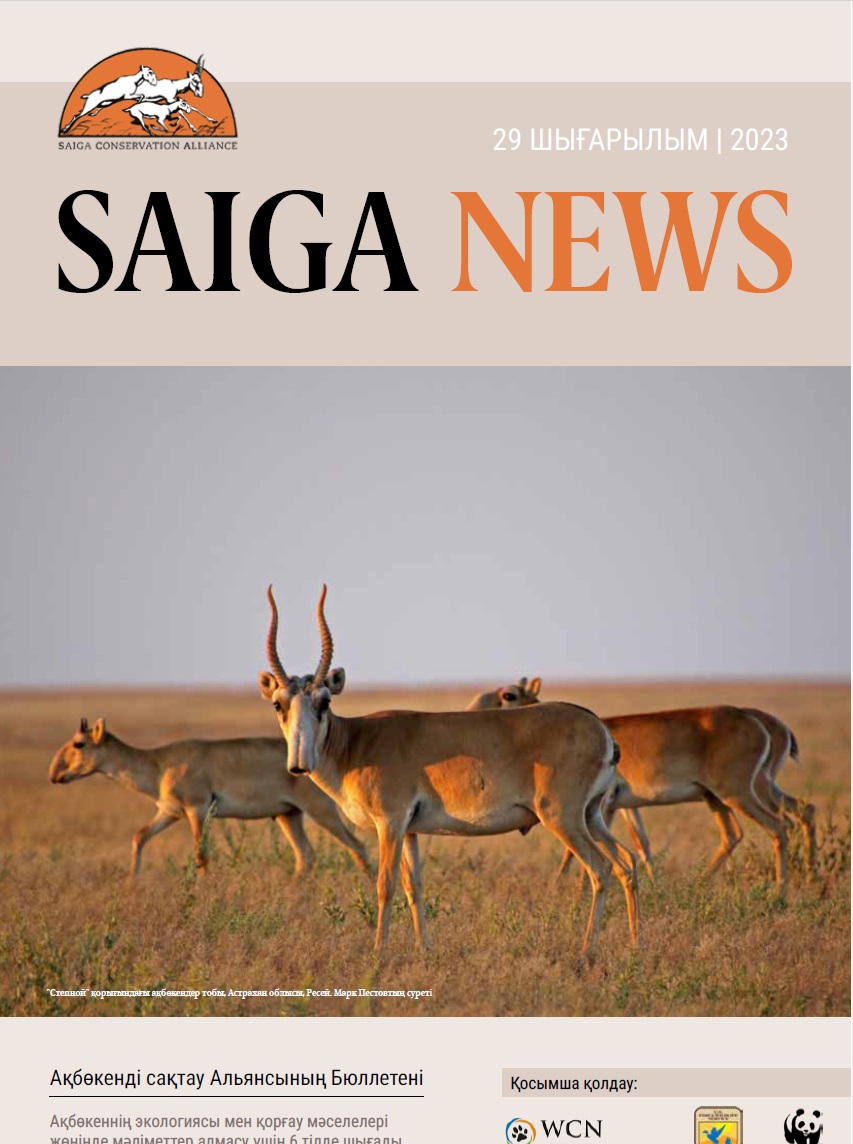The cover of the magazine or newsletter features a light tan background at the top and bottom. In the upper left corner, a logo resembling an orange half-sun filled with white antelope silhouettes represents the Saiga Conservation Alliance. To the right, the date "29 [Month in another language] 2023" is displayed in white text. Beneath this, the title "Saiga News" is prominently presented, with "Saiga" in large black letters and "News" in orange. The central portion of the cover is dominated by a color photograph of three tan-colored antelopes with white faces. The antelope in the foreground, which has curvy antlers, faces the camera, while the two others, without antlers, are oriented to the left. All three are standing in brown grass, possibly captured during a sunset, given the warm illumination. The photograph has a white caption in another language at the bottom. Logos for WCN and the World Wildlife Fund, featuring the iconic panda, are positioned at the bottom right corner.